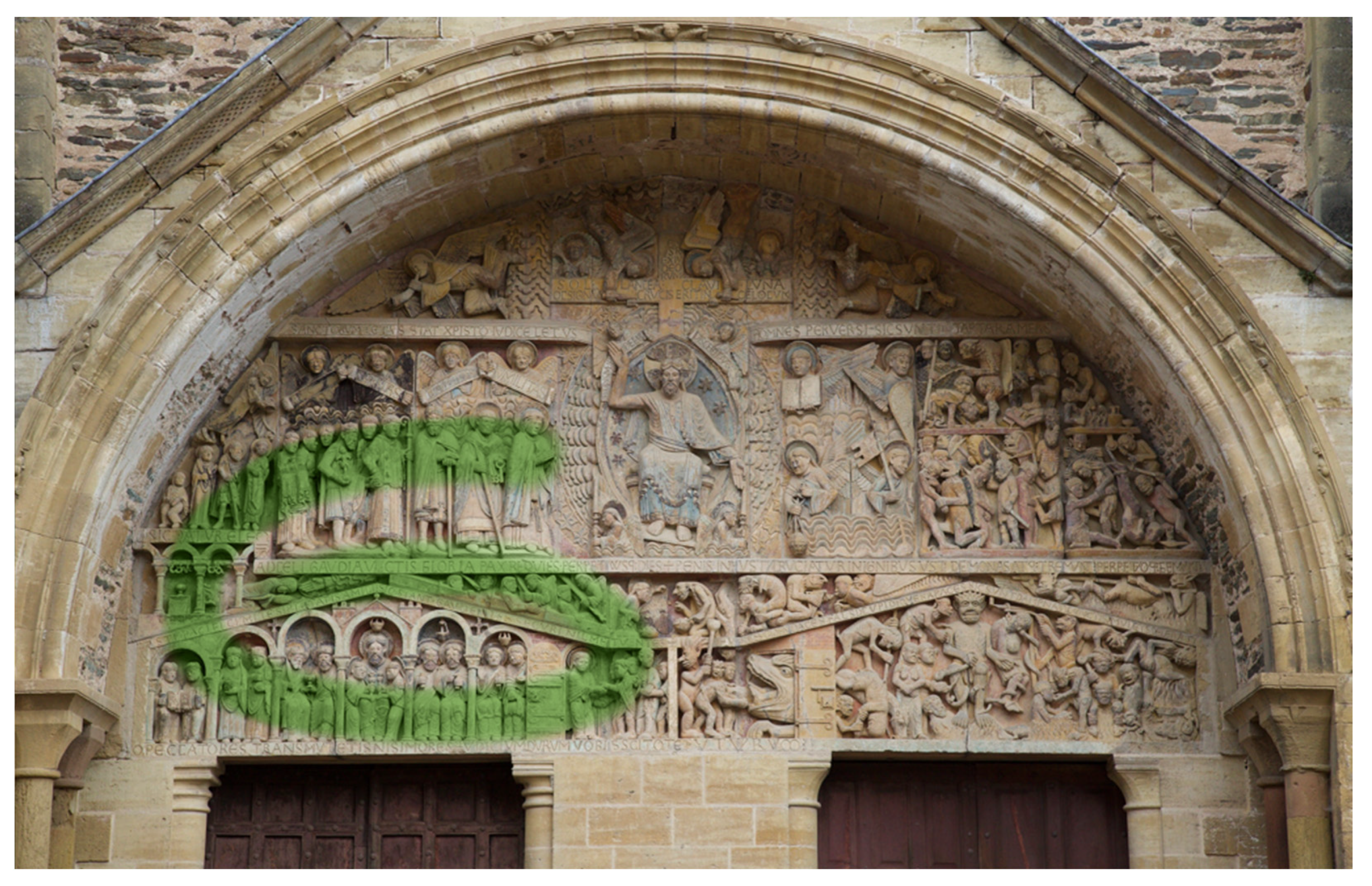This photograph captures the ornate arched entryway of an ancient building, possibly a church or a historic site, characterized by intricate stone carvings. The beige-colored stonework forms an arch that frames the upper part of wooden, hand-carved doors. Prominently, a lower and upper relief adorns the arch, divided into three sections, meticulously detailed with figures in various poses and scenes.

The central section hosts a dominant religious figure, seemingly Jesus, discernible by the halo behind his head. He stands with one hand raised and the other by his side, clothed in a simple robe. Surrounding him are a multitude of figures, including angels, cherubs, and worshippers, some of whom are holding open bibles or symbols of faith. Above this central figure, the topmost section depicts what looks like people falling amidst celestial scenes, possibly accompanied by flutists.

The carvings on the left side of the arch portray an organized line of standing individuals, while the right side features a more chaotic cluster of figures. Below these, the scenes continue with people sitting and interacting, representing a mix of men, children, and even some animals within the carvings. This area is dense with history, telling tales of battles, sexuality, and community life from its society's past.

Notably, the archway has been marred by modern interference, with a green spray-painted letter 'G' visible on the left side of the frieze, juxtaposing harshly against the aged, mossy surface of the stone. Despite this blemish, the artistry of the relief remains a vibrant historical testament to the building's storied past.